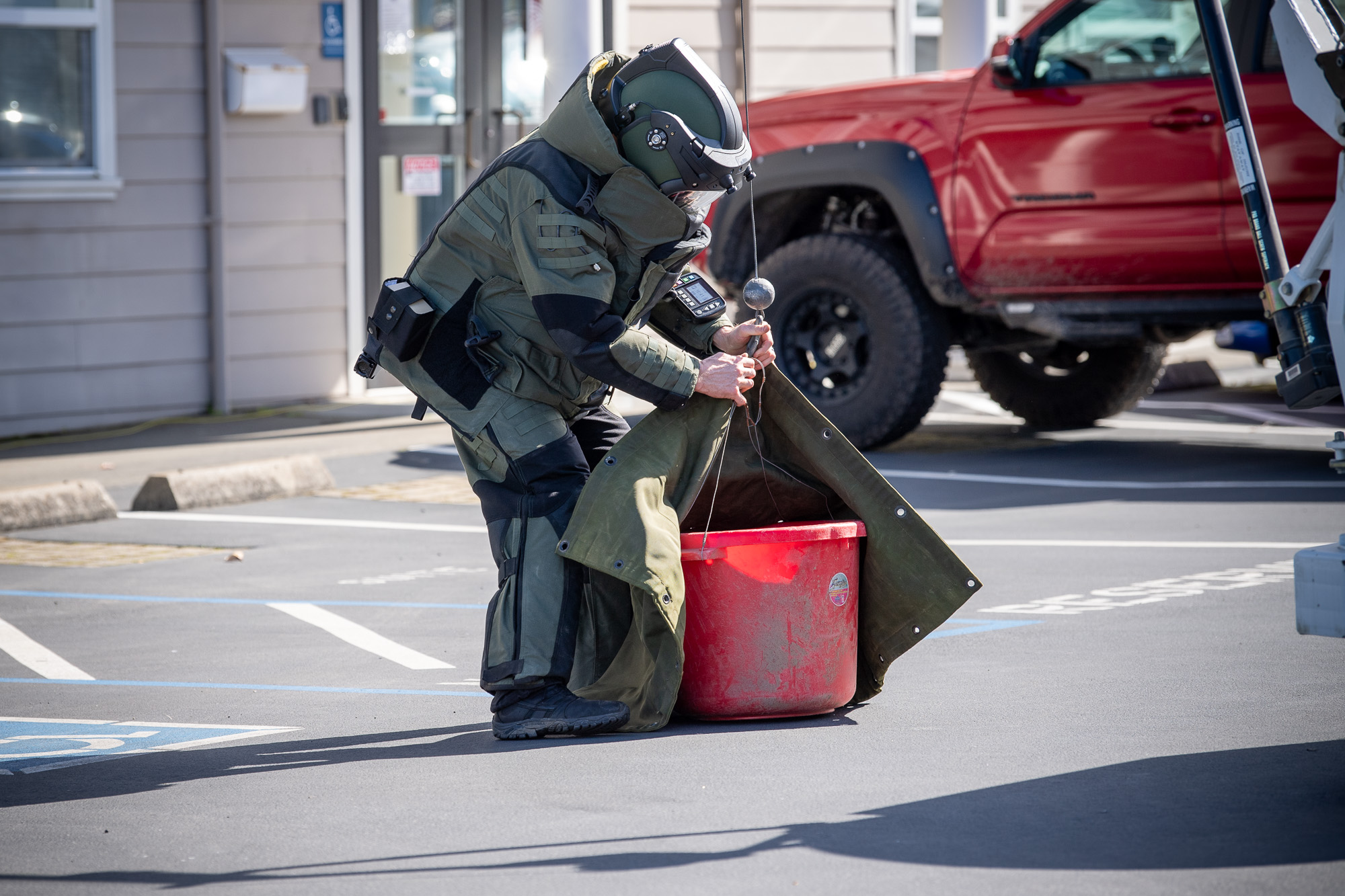In the image, a person dressed in a full bomb disposal suit, which includes a military-style helmet, jacket, and pants, is standing in a gray asphalt parking lot during the daytime. The person, possibly a member of a bomb squad, is handling a red container box, wrapping it with a thick cloth or military bag, possibly to contain or retrieve the contents safely. Despite being covered from head to toe, their bare hands are visible. To their left arm, a small monitor with numerous buttons is visible, and on their right hip, there's a noticeable black box. In the background on the right side, there's a large red utility truck with black tires, black fenders with rivets, and an elevator platform. Adjacent to this scene, on the left, stands a beige building with two central, black double doors and white-framed windows. Several handicapped parking spaces, marked with blue and white designs, are also visible in the parking lot. The scene suggests a mix of colors, prominently featuring green, red, beige, and gray. The overall impression is one of a meticulous practice or rehearsal, potentially for bomb disposal or emergency response scenarios.